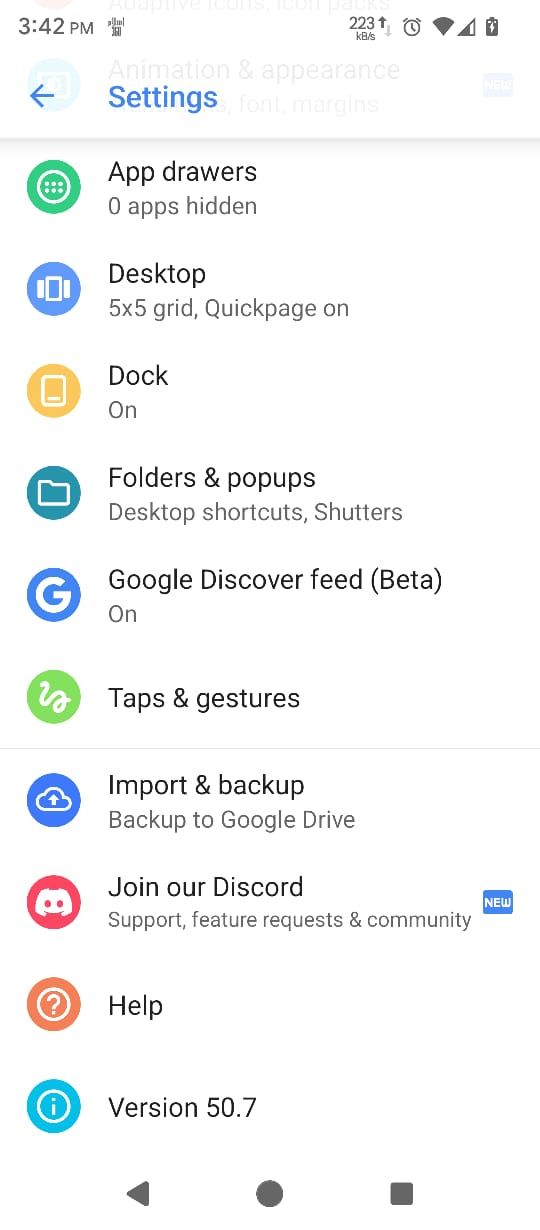This image depicts a screenshot from a mobile device, most likely a phone, as suggested by the aspect ratio and the typical status indicators at the top of the screen. These indicators include a battery icon, Wi-Fi symbol, and a signal strength icon, with the current time displayed as 3:42 PM. 

The primary portion of the screen shows a settings menu with a white background and black text. The settings categories are presented in a list format, each with a colorful icon to the left. The icons feature various colors such as blue, yellow, and green, which stand out against the otherwise monochromatic theme of the page. 

Here are the settings categories listed:
- App Drawers
- Desktop
- Dock
- Folders and Pop-ups
- Google Discover Feed
- Taps and Gestures
- Import and Backup
- Join Our Discord
- Help 
- Version 50.7

Additionally, at the bottom of the screen, the familiar navigation icons typical of Android devices—back, home, and recent apps—are visible. This detailed settings menu allows users to customize various aspects of their device.